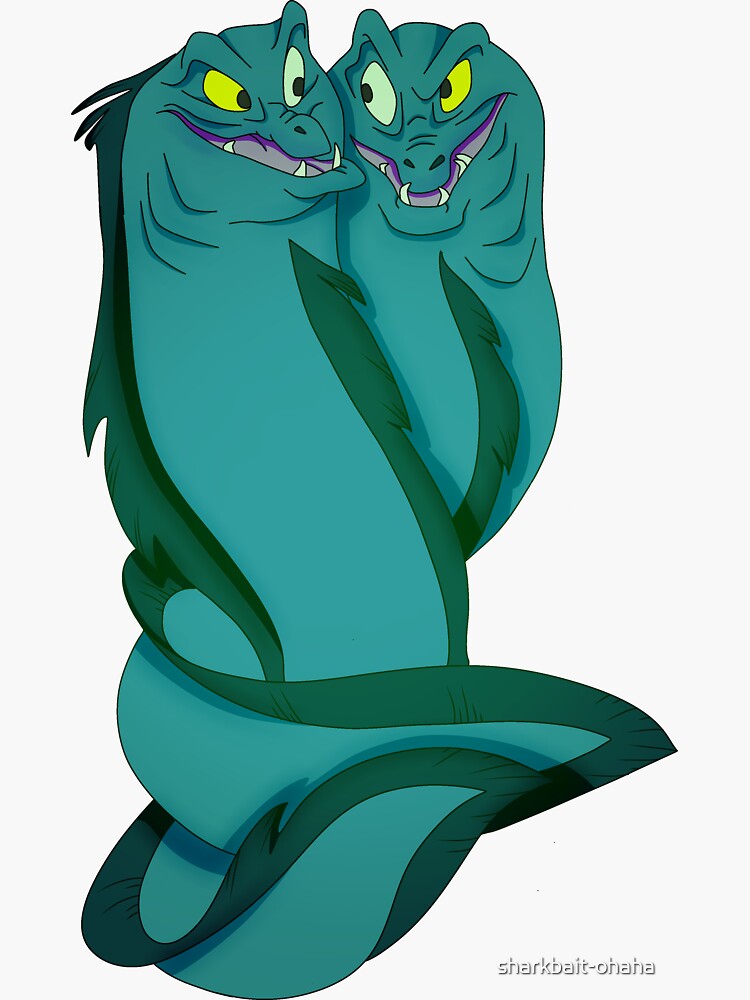The illustration depicts two identical, intertwined cartoon creatures with a striking resemblance to the moray eels from Disney's "The Little Mermaid." Their serpentine bodies are a teal green color with darker green fins resembling manes running along the top and bottom. They lack arms and legs, ending in mermaid-like tails that curl around each other. Their vicious expressions are highlighted by open mouths displaying pointed teeth or fangs, with the insides of their mouths tinged purple. The creatures possess two different color eyes—one golden and one light blue—adding to their menacing appearance. They fiercely glare at each other, suggesting an imminent clash. At the bottom of the poster, the text "Sharkbait-Ohaha" is displayed, though no further explanation is provided.